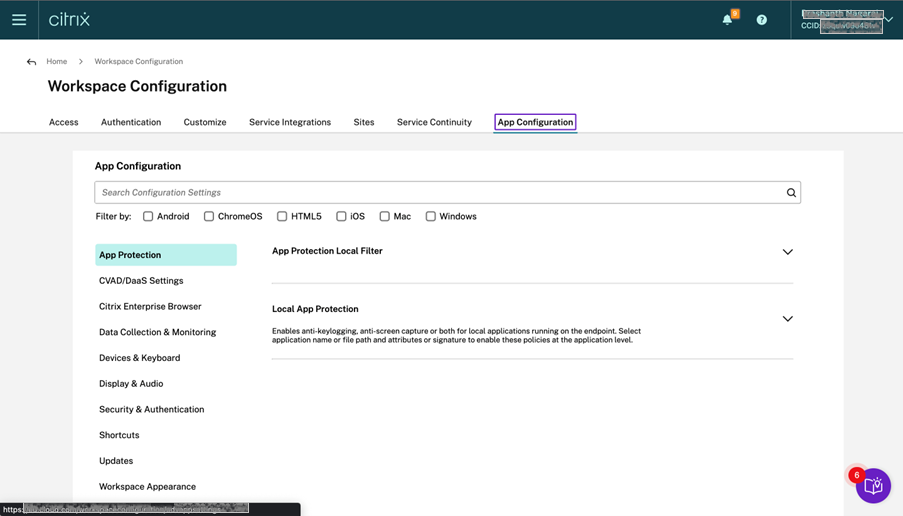The image showcases a Citrix website interface. At the top, there is a thin black banner stretching across the page. On the far left of the banner, there is a recognizable "hamburger" menu icon composed of three horizontal lines, next to the "Citrix" logo, both in a light blue font. Moving rightward on the banner, there are several small icons including an alert symbol, marked with a red notification indicator in the upper right corner, and a question mark icon. Adjacent to these icons, there is a readable dropdown menu, albeit in small, outlined text.

Below this banner, on the left, there is a breadcrumb navigation trail in small text, indicating "Home > Workspace Configuration." Directly below this, in a larger and bolder font, the title "Workspace Configuration" is displayed. Further down, the interface features seven tab options extending horizontally to the right, with the "App Configuration" tab highlighted by a purple outline.

The main content area beneath these tabs consists of a gray background with a prominent white box centered within it. Inside this box, the header "App Configuration" is visible, alongside a text box designed for searching different settings. Below the search box, there are filter options including checkboxes for "Android" and "Chrome OS."

Subsequently, various selectable options are listed vertically, such as "App Protection," "Citrix Enterprise Browser," and "Data Collection Monitoring." The "App Protection" option is chosen, indicated by a light blue highlight. To the right of this, detailed text explanations for "App Protection Local Filter" are visible, accompanied by a dropdown arrow for additional options.

Overall, the website's layout is structured, with clear sections for navigation, configuration, and detailed settings for Citrix workspace management.